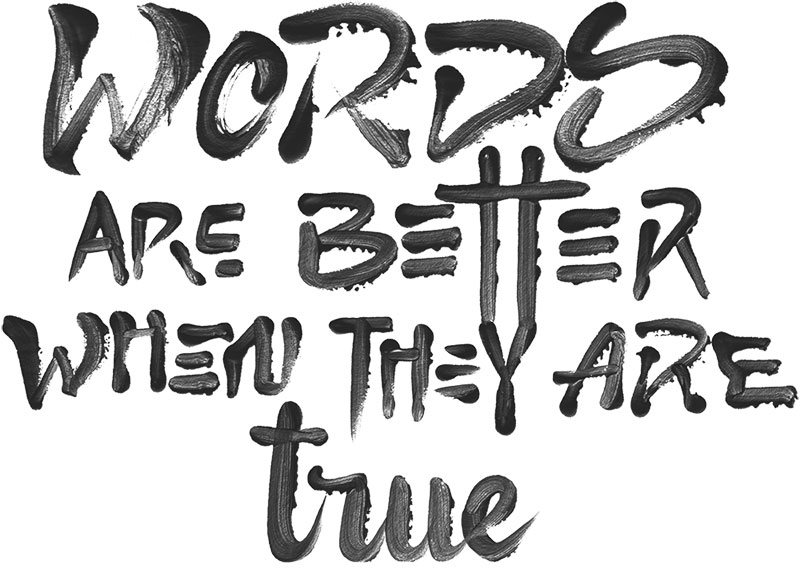The image features a poster with a simple yet impactful design: black text on a white background. The text reads, "Words are better when they are true," and it appears to have been applied with a paintbrush, evident from visible brush strokes and occasional drip marks. The layout is divided into four lines: "WORDS" on the first line, "ARE BETTER" on the second, "WHEN THEY ARE" on the third, and finally "TRUE" on the fourth. The word "WORDS" is in all uppercase letters, as is "ARE." The word "BETTER" is also in uppercase, but the two 'T's are distinctively connected by a single horizontal line. The letters 'E' in "BETTER," "WHEN," and "THEY" are uniquely represented by three horizontal lines each, lacking the vertical stroke. The final word, "TRUE," stands out in neat cursive, contrasting the previous block-like text. This combination of varied styles highlights the message's emphasis on authenticity.